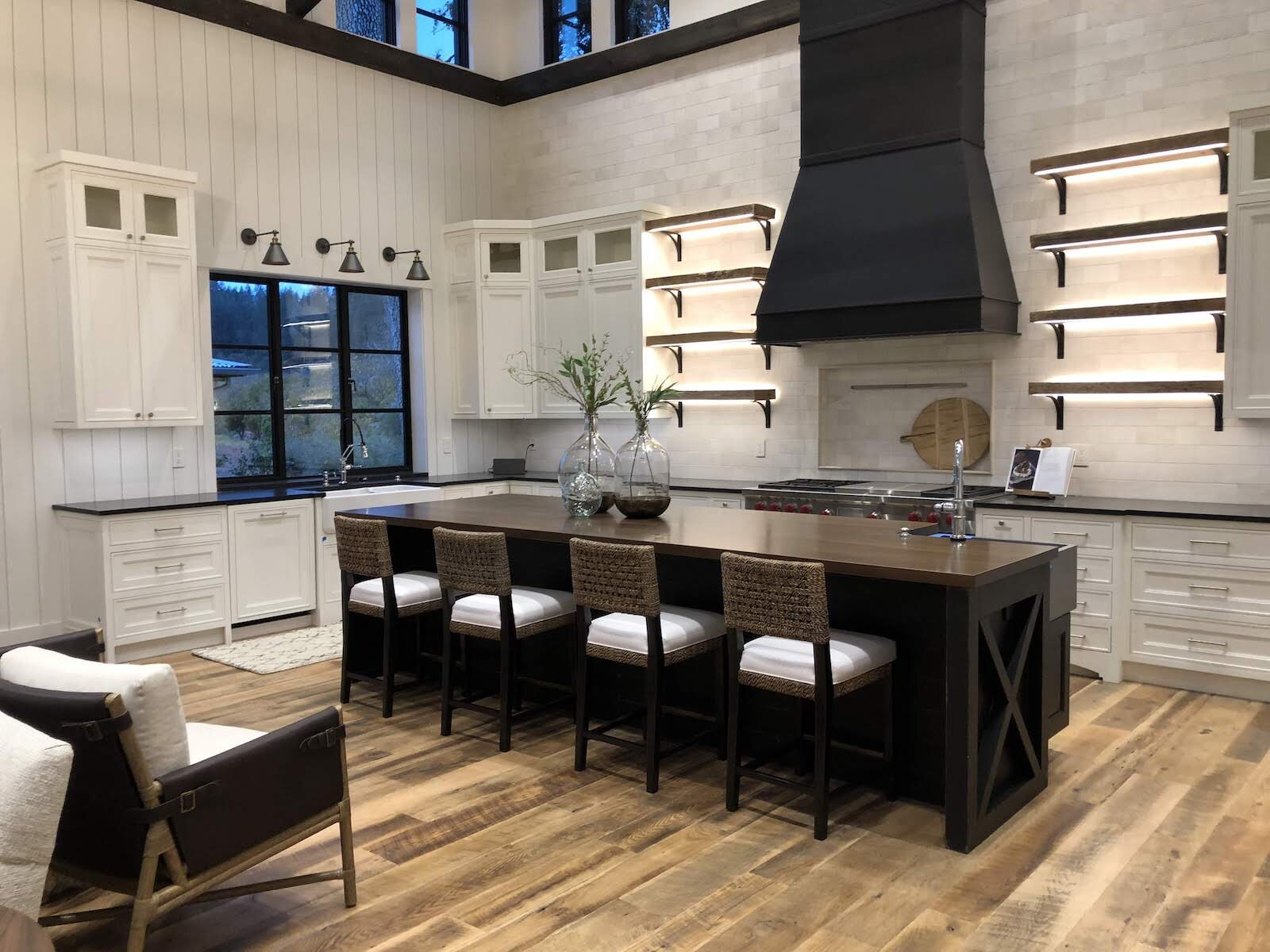This photograph showcases a stylish and modern kitchen-dining area within a home, likely staged for a real estate listing. At the center of the image is a large dark wood kitchen island serving as the main focal point. The island features an attached sink on the far side and is surrounded by four high wicker chairs with white cushions, lined up along the near side. The seating points towards the kitchen, creating a welcoming ambiance for gatherings.

The background reveals a well-equipped kitchen with a black granite countertop. The cooking area includes a range with an oven, topped by a prominent black exhaust hood. Flanking the hood are two shelving units illuminated by integrated lights, adding a warm glow to the space. White, country-style cabinets extend across the kitchen, complemented by a silver sink under a window with a paned design, suggesting a blend of modern and traditional aesthetics.

The room's rich hardwood floors harmonize with the island's dark wood, while an upholstered armchair with white cushions is positioned behind the island, adding a touch of comfort. The overall scene is one of elegance and functionality, with subtle details that make the space feel both inviting and luxurious. The presence of a mezzanine or partial second floor above the kitchen adds architectural interest to the overall design.